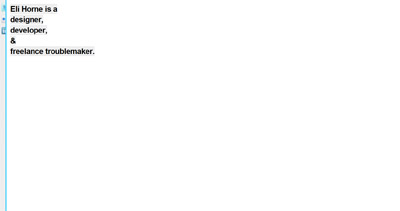In the image, there is a white page featuring black text that reads, "Eli Holm is a designer, developer, and freelance troublemaker." To the left of this text is a vertical blue strip, which adds a splash of color to the otherwise monochromatic layout. The clean and minimalistic design emphasizes the textual content, creating a striking contrast between the black letters and the white background. This page appears to be part of a portfolio or personal introduction, showcasing Eli Holm's professional roles and playful personality.